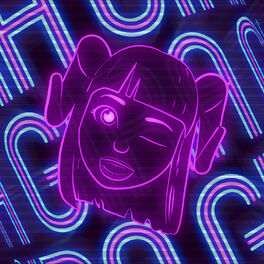This square piece of artwork features a cartoon-style character that resembles an anime or Japanese cartoon figure. The central focus is on a head of possibly a young woman or girl with upper neck-length hair and bangs. Her hair and face are predominantly shaded in black, highlighted with neon purple-pink to create an impression of neon lighting. She sports curled ram-like horns on the sides of her head. One of her eyes is open while the other is winking, and she has an open mouth with a slight smile. Her expression is accentuated by one slightly raised eyebrow. The background is solid black, overlaid with glowing neon text in purple and fluorescent blue. The text appears to consist of repeated, fragmented letters such as G, H, and A, but does not form any discernible words due to the image's close-up focus.